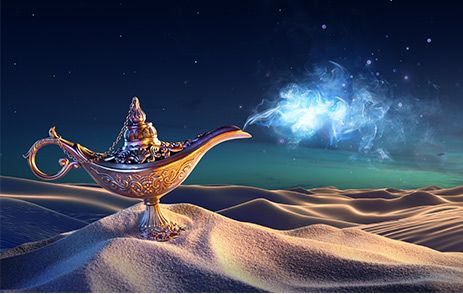This is a smaller horizontally aligned rectangular, AI-generated image. The top portion features a solid black starry night sky, which transitions into dark blue, and eventually into a light teal, representing ocean water. Beneath the water lies an expanse of light beige sand dunes with detailed grain visible in the foreground. Positioned on the left side of the sand is a gold-colored magic genie lamp with a circular handle on the left and a spout on the right. Emerging from the spout is a white, cloud-like puff of smoke. The overall scene blends elements of a surreal landscape with fantastical elements, creating a strikingly unique visual.